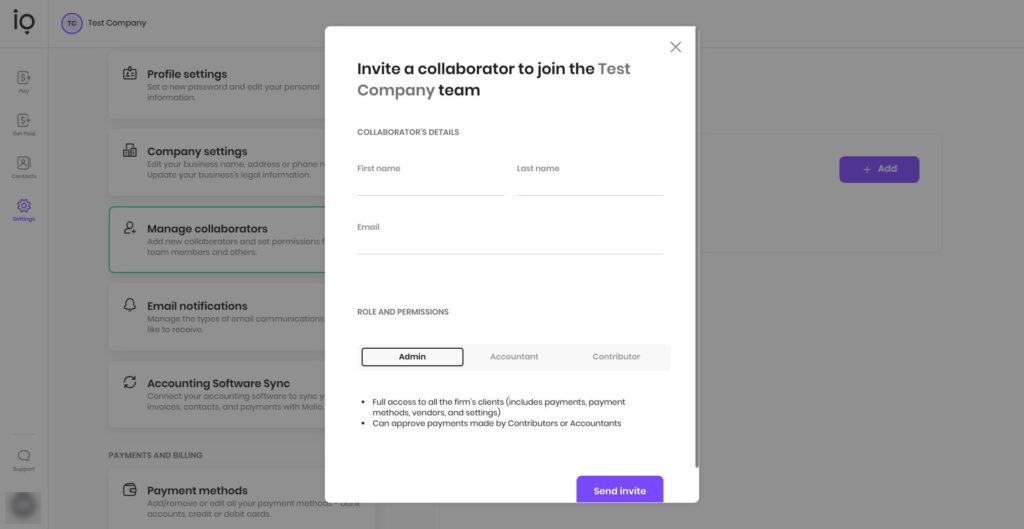This is a detailed screenshot of a web page with a prominent vertical inset overlay that partially obscures the main content. In the upper-left corner of the main page, there is a logo that reads "I O" with a triangle pointing down beneath the 'O'. To the right, there's a purple circle bearing the initials 'TC'. Next to this, the text "Test Company" appears twice in a row.

The main page features several categories listed sequentially:
1. **Profile Settings**: Allows users to set a new profile, among other options.
2. **Company Settings**: Enables editing of business name and other details.
3. **Manage Collaborators**: This category is highlighted with a green outline and includes options to add new collaborators and more.
4. **Email Notifications**: Facilitates the management of various email communications.
5. **Accounting Software Sync**: Provides options to connect your accounting software.
6. **Payments and Billings**: Follows under a distinct headline called "Accounting".
7. **Payment Methods**: Here, users can add, remove, or edit their payment methods.

On the far-left sidebar, there are four tabs:
1. **Pay**
2. **[Illegible]**
3. **Customize (possibly)**
4. **Settings**

The inset overlay, which is highlighted from the "Manage Collaborators" section, is a white, vertical rectangular box. It includes text inviting a collaborator to join "Test Company", with "Test Company" written in dark gray and the rest in black. The text "Test Company Team" is also present. 

Below this, there are fields for entering the collaborator's first name, last name, and email. There is a section titled "Role and Permissions," with three categories:
1. **Admin**: Highlighted with a black bar, this role offers full access to the firm's clients and allows for approval of payments made by contributors, among other privileges.
2. **Accountant**
3. **Contributor**

At the bottom of the inset, there is a prominent purple "Send Invite" button.